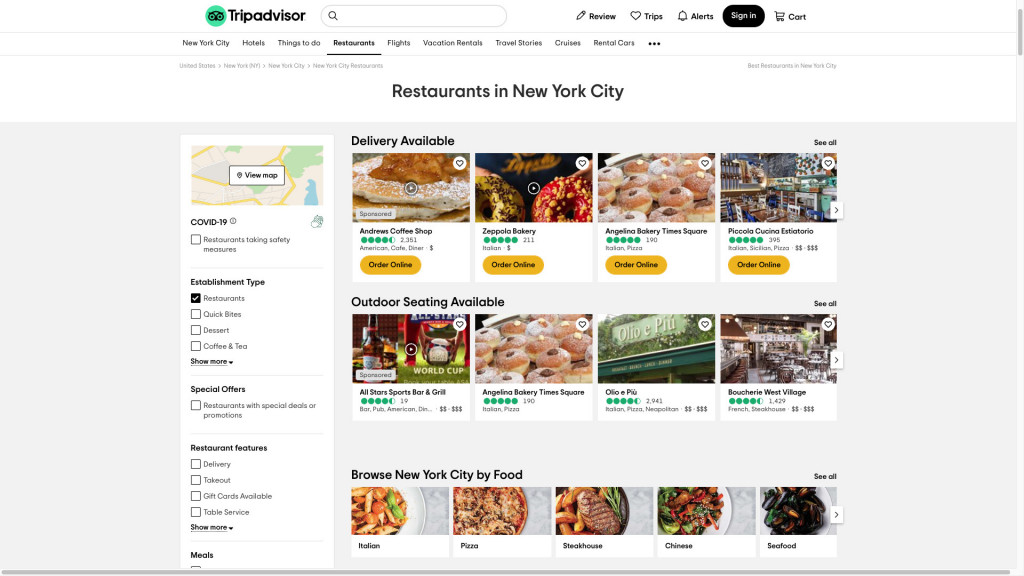This image showcases the TripAdvisor website, a comprehensive platform where users can find detailed information about hotels, restaurants, flights, vacation rentals, travel stories, cruises, and rental cars for any city in the world. Dominating the top of the webpage is the TripAdvisor logo, depicted as a green circle with a stylized owl's face. Directly beneath the logo lies an efficient search bar. 

The specific webpage displayed focuses on restaurants in New York City. Users are presented with several options, displayed at a rate of four entries per row. The first row highlights restaurants that offer delivery services, featuring venues such as Andrew's Coffee Shop, Zappola Bakery, Angelina Bakery Times Square, and Piccola Cucina Estatorio. Each restaurant's entry includes a mouth-watering photograph of their popular dishes, the establishment's name, its rating out of five stars, and the total number of reviewers who have rated the restaurant.